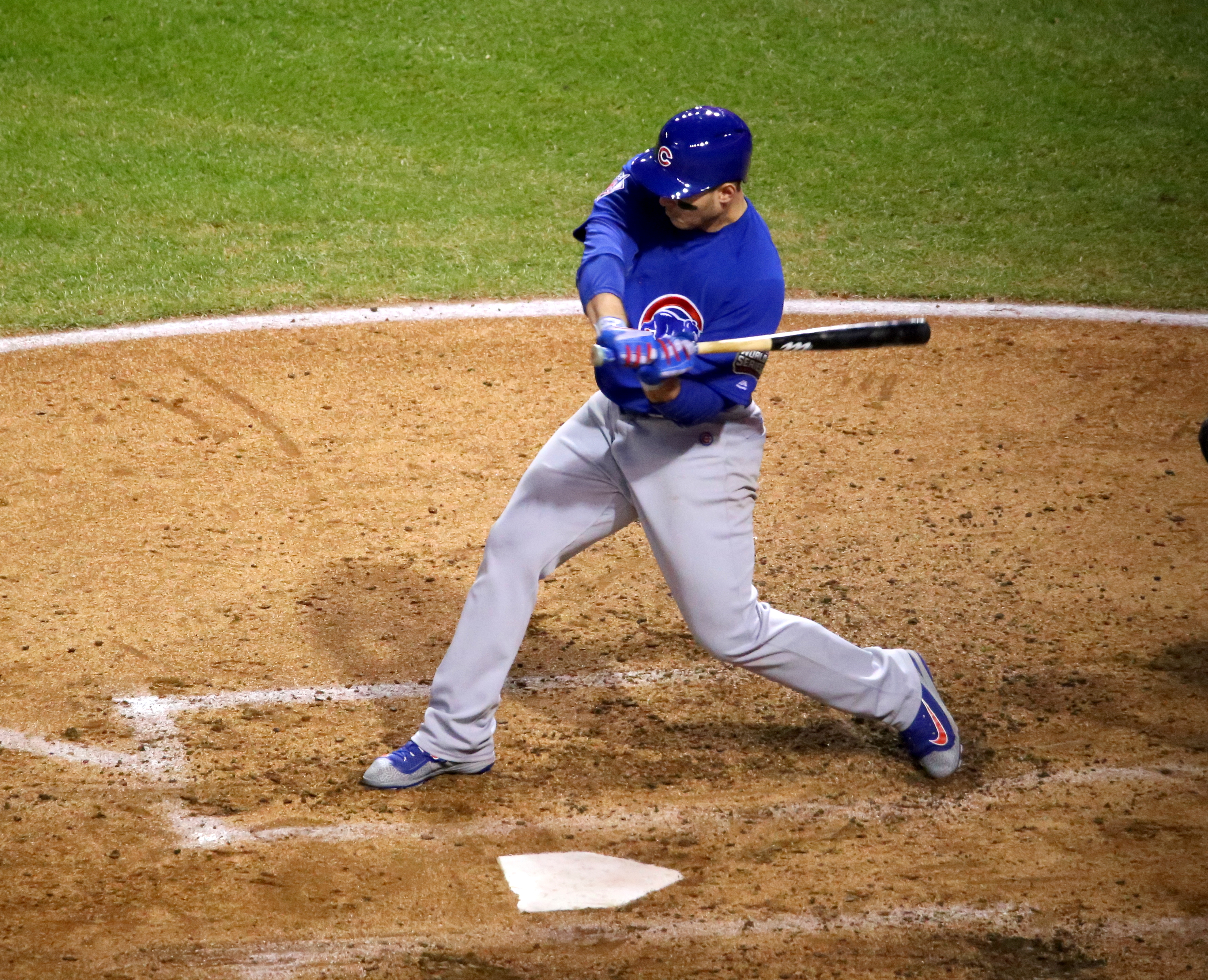The image captures a dynamic moment of a baseball game, focusing solely on the batter who is mid-swing. The photograph shows the player from a side angle, with his body slightly turned toward the camera. His left leg is bent at the knee, while his right foot is more straight, indicating his twisting motion to generate power. The bat, held near his chest, appears blurry, emphasizing the speed of the swing. He stands on a well-trodden brown dirt area near the home plate, with some green grass visible beside it.

The player's uniform is distinctive: a blue short-sleeved shirt with a red "C" partially obscured by his hands and bat, an illustration of a bear indicating it's the Cubs team; grey pants; blue and grey shoes; and a blue helmet also marked with a red "C." The helmet obscures much of his face, showing only white or slightly tan skin, suggesting he could be Hispanic or white. The field also features visible chalk outlines on the grass, enhancing the authenticity of the baseball setting.